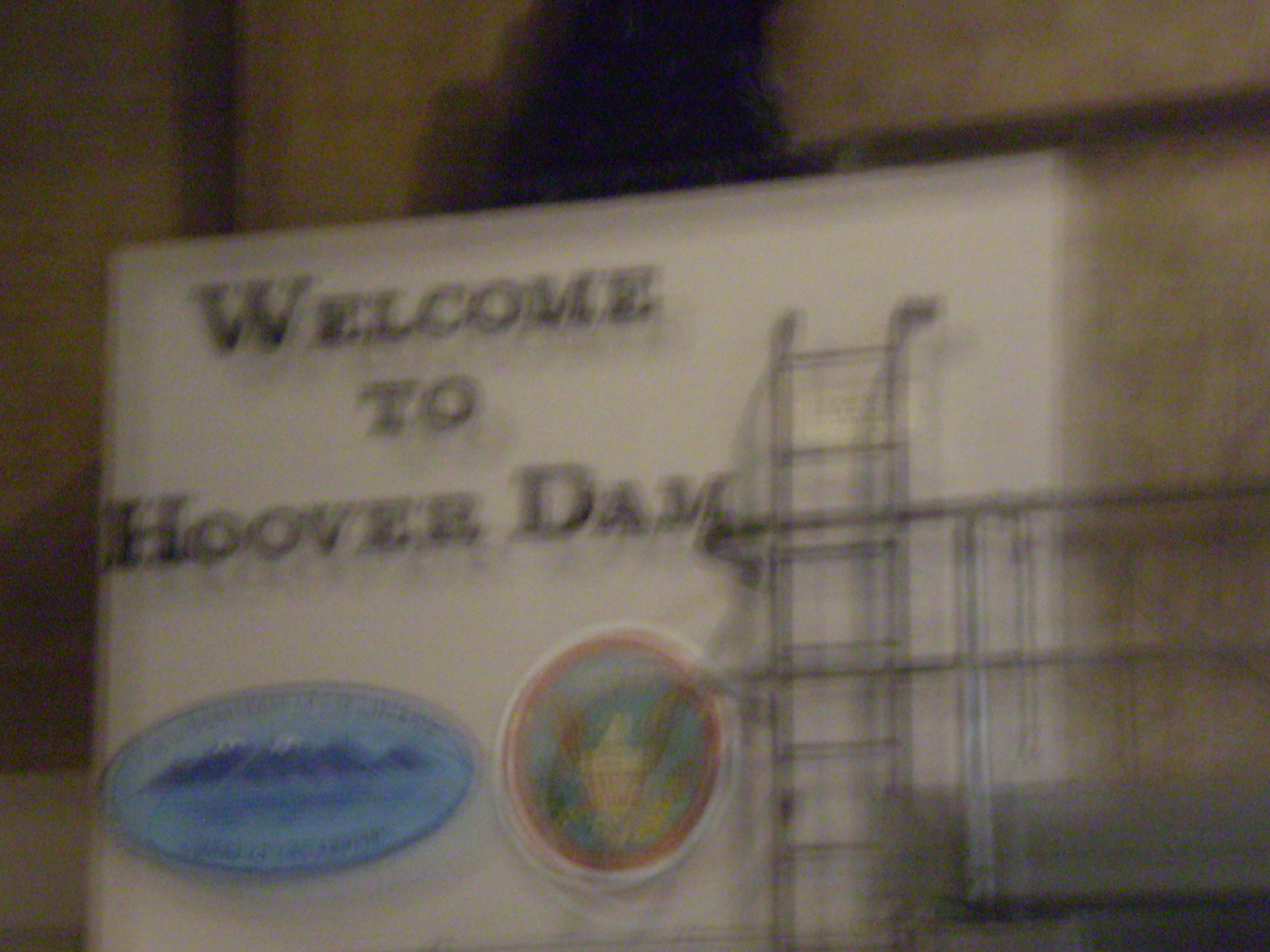The image depicts a slightly blurry photograph of a white sign with bold black lettering that reads "Welcome" on the first line, "to" on the second line, and "Hoover Dam" on the third line. Below this text, there's a horizontally elongated blue oval label that appears to feature a mountain with snowy ice caps. To the right of this blue oval is a vertically oriented circular emblem which seems to depict an eagle holding items in its talons, likely on a blue background, bordered by a red and then a white outline. To the right of the sign, there is visible scaffolding and a ladder. The background of the image consists of what looks like a tan concrete wall. Despite the blurriness, these details are discernable.